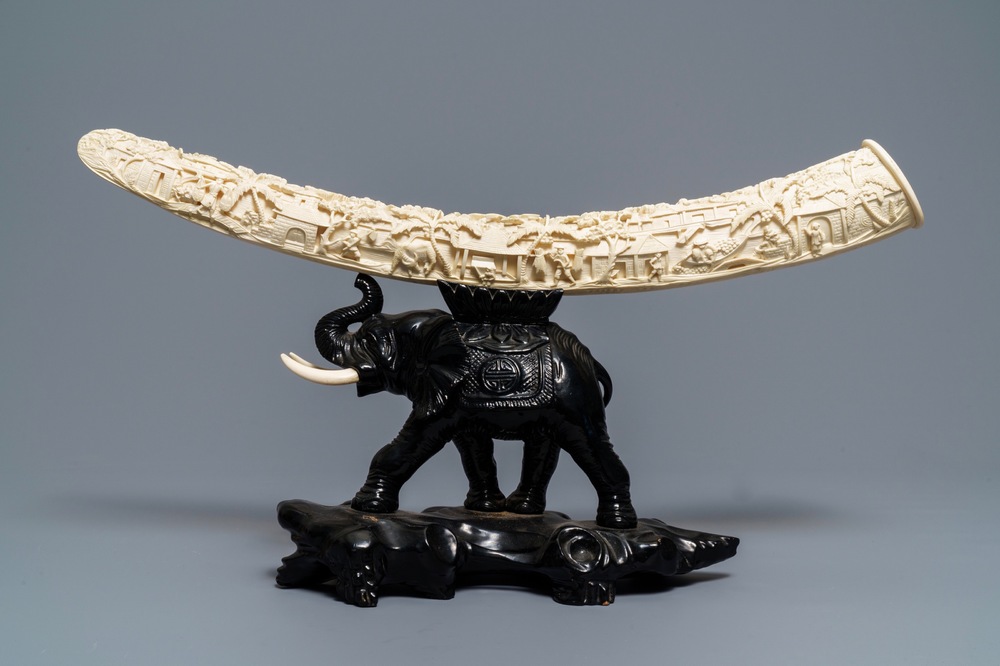In this detailed image, a black marble carving of an elephant takes center stage against a light blue background. The elephant, facing the left with its trunk curled upward, showcases two prominent white tusks extending to the left. Delicately carved details adorn the elephant, including a blanket-like design on its back and a platform that supports an intricately designed arc. This arc, also white, is longer than the statue itself and features various elaborate carvings, such as palm trees. The elephant stands atop a glossy black base, which could be another figure or simply a rock stand, contributing to the sculpture's overall elegance and complexity.